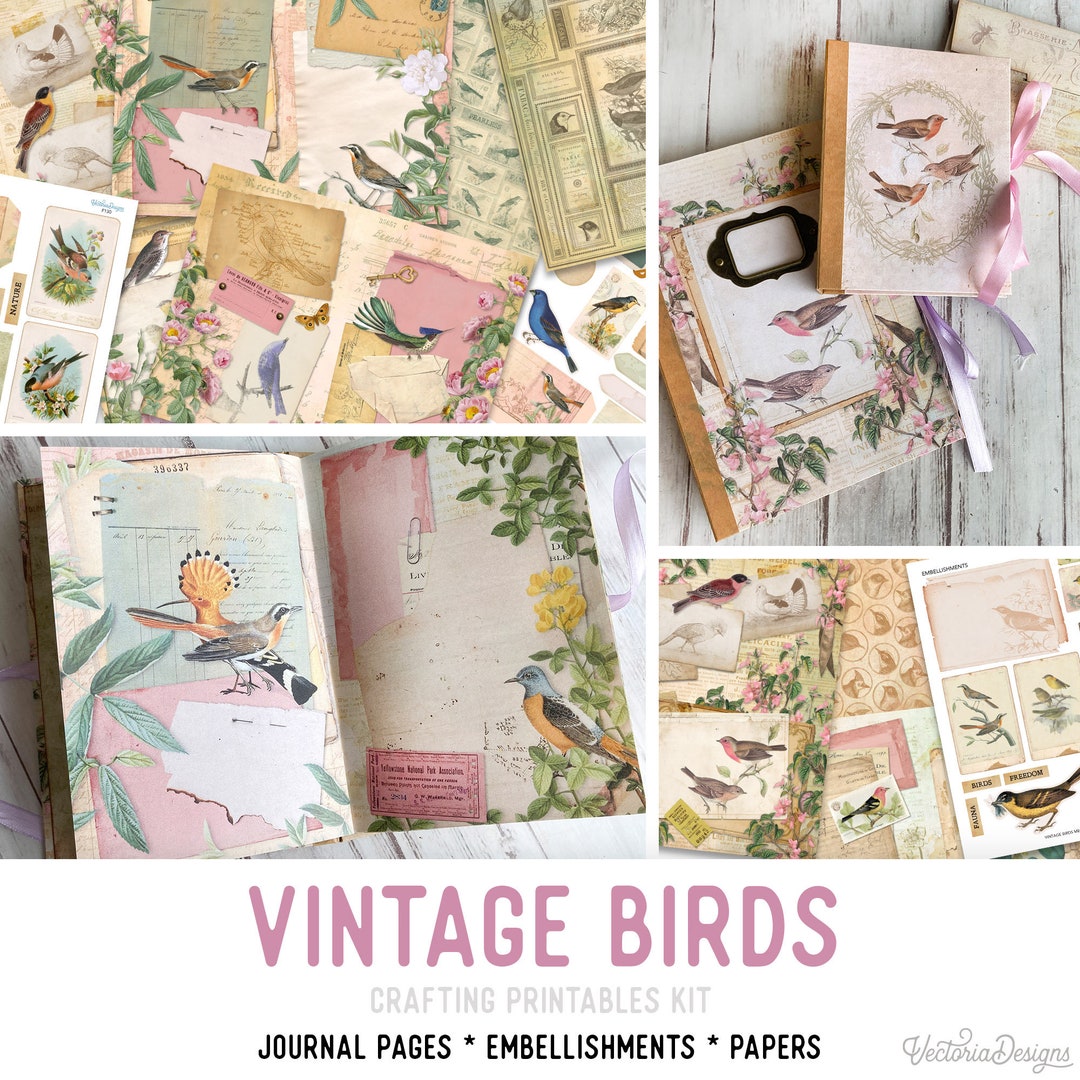The image is a slightly taller-than-wide collage featuring four distinct sections, each depicting elements from the "Vintage Birds Crafting Printables Kit" by Victoria Designs. At the bottom, against a white background, the text "Vintage Birds" is elegantly written in pink, followed by gray and black subtext reading "crafting printables kit, journal pages, embellishments, papers." A logo signature of Victoria Designs is placed in the lower right corner.

The upper left section displays a collection of decorative postcards or papers adorned with illustrations of various birds and lush vegetation. The upper right section showcases a box, also featuring bird and floral designs, possibly a cover for a book like a diary, embellished with ribbons in pink and purple. The lower left section portrays the open pages of a book, whimsically detailed with the same bird and plant motifs, suggesting its use as a journal. Finally, the lower right section presents what seems to be stickers or labels, continuing the theme with intricate bird and flower imagery.